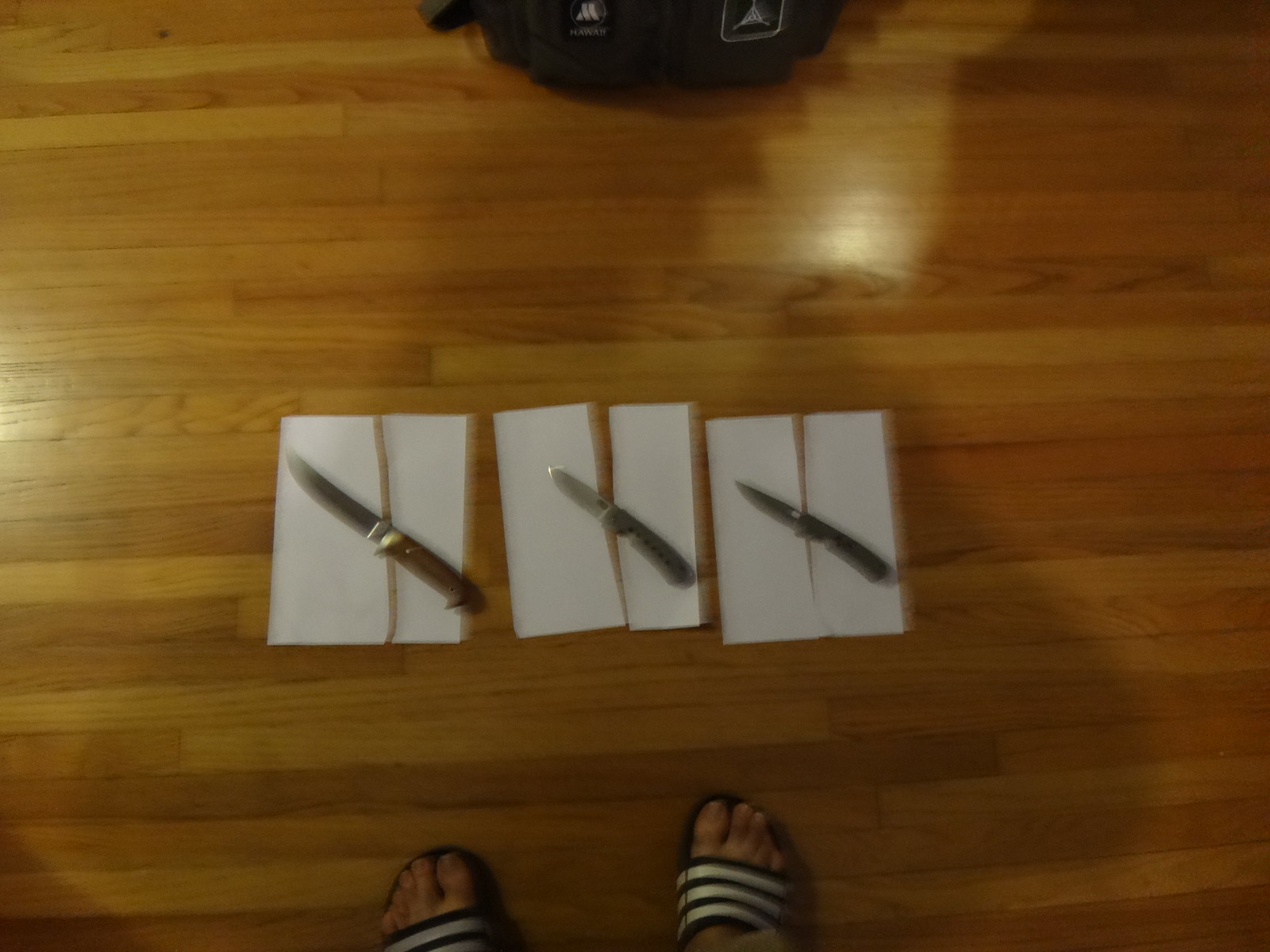This slightly blurry, overhead photograph captures a detailed scene on a reflective, golden tan wooden floor, characterized by thin, elongated planks. At the bottom center of the image, there are two feet clad in black slides with white horizontal stripes, possibly Adidas sandals, displaying the toes of the photographer. The focus of the image is the center where three slices of white paper, cut diagonally into six pieces, are laid out. Each pair of sliced paper sections is topped with a different knife, all positioned diagonally with the blades pointing toward the top left corner and the handles toward the bottom right. The leftmost knife, with a large wooden handle, is the biggest, followed by a smaller knife in the center with a shorter blade, and the third knife on the right with a pointed blade and dark handle. Above these papers, at the top center, part of a black object, perhaps a bag or backpack, is just visible, adorned with a few white logos. The scene is bathed in varied lighting, creating numerous shadows across the floor and papers, with the left edge of the photo appearing brighter than the right, and a bright spot noticeable between the black object and the papers.